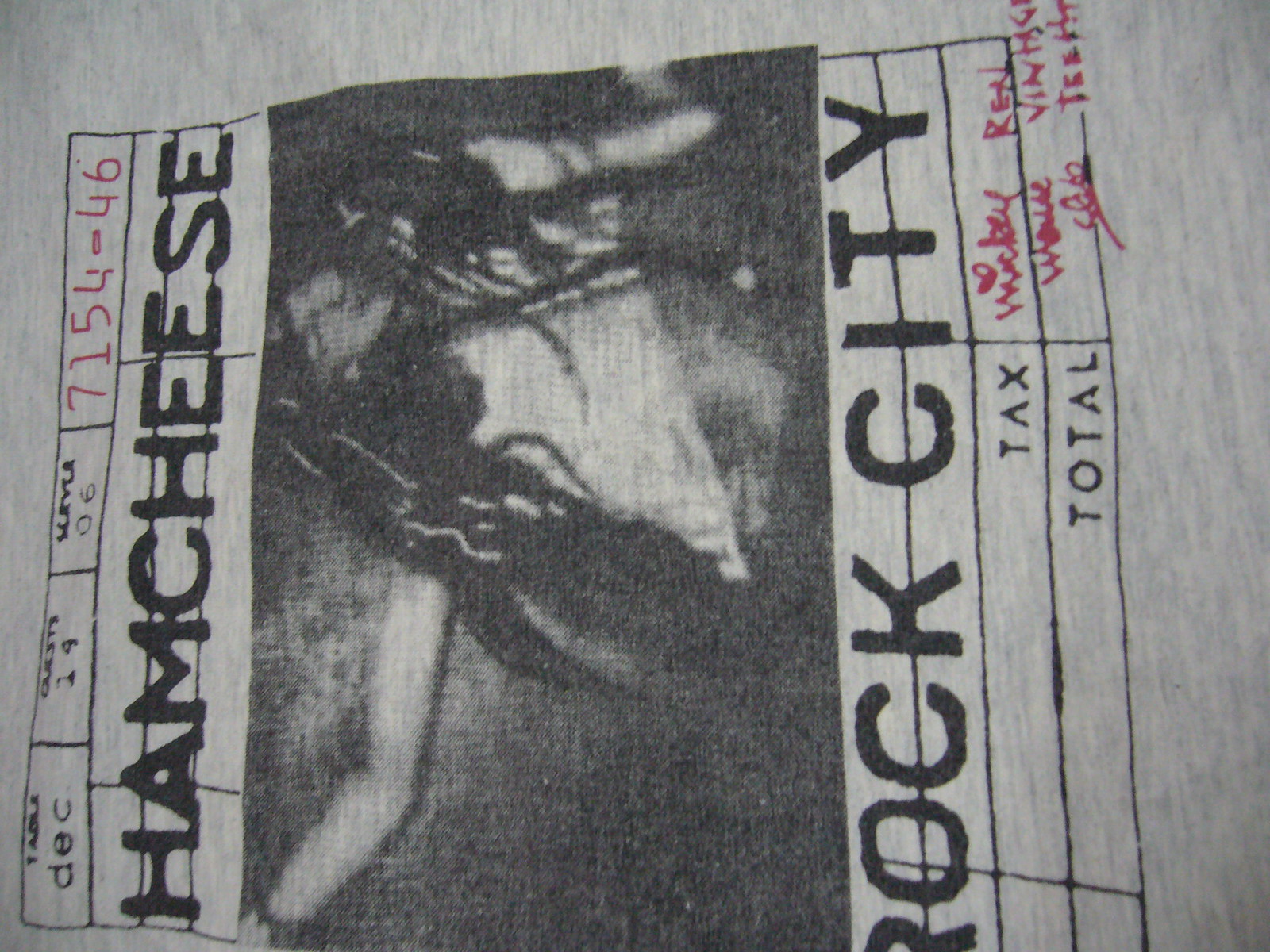The image depicts a t-shirt featuring a possible band or concert graphic, displayed at an angle. At the top of the t-shirt, it reads "December 14, '06." Below that, the text "7154-46" is written in red letters. The main graphic element showcases the phrase "Ham, Cheese, Rock, City" also in red text. Scattered around this text are additional red writings that appear to be signatures. Centrally placed on the t-shirt is a grainy black and white photograph of a person with long hair, wearing a white tank top, set against a dark background. The overall design gives the impression of a vintage concert souvenir.